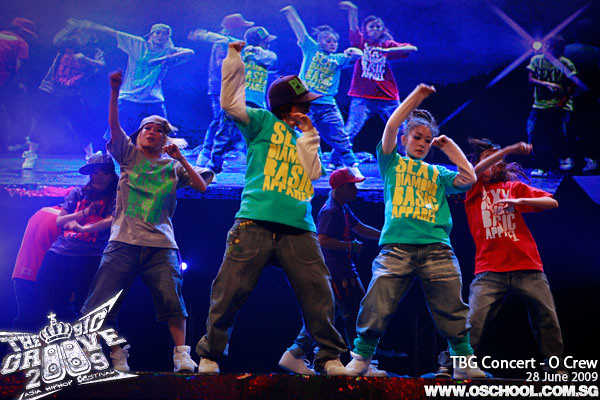The image depicts an indoor club event with several young children dancing on a stage under spotlights in a dark environment. The children are in mid-pose, arms raised and legs wide apart, as if performing a dance move. On the far right, a child wears a red t-shirt with white text and gray pants. Next to him, a girl in a green t-shirt with yellow text and gray pants stands beside a boy in a similar green shirt with yellow text and gray pants, both donning baseball caps. To their left, another girl in a gray shirt with green text and blue capri pants also sports a baseball cap. Altogether, around seven or eight children are dancing, with four wearing hats. The scene is enhanced by various colored lights around them, mainly purples and blues. In the background, a large screen shows the children dancing. The bottom of the image features white text: on the left, "The Big Groove 2009"; on the right, "TBG Concert-O Crew, 28 June 2009, www.oschool.com.sg".